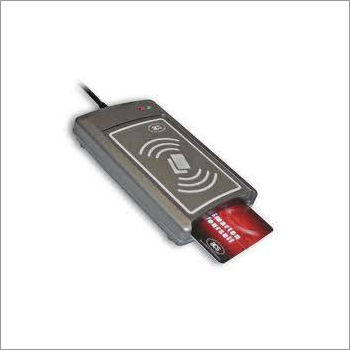The image features a gray card reader positioned diagonally from the top left to the bottom right against a stark white background with a very thin border. A short black cord extends from the top left of the card reader, which also has a pair of inactive red and green lights on its top right corner. The center of the card reader displays a label with a symbol of two cards overlaid with curved lines above and below them, all outlined in white. A red, white, and black card is partially inserted into the bottom of the card reader. The image presents a clean, simple, and detailed product shot, emphasizing the modern and functional design of the card reader.